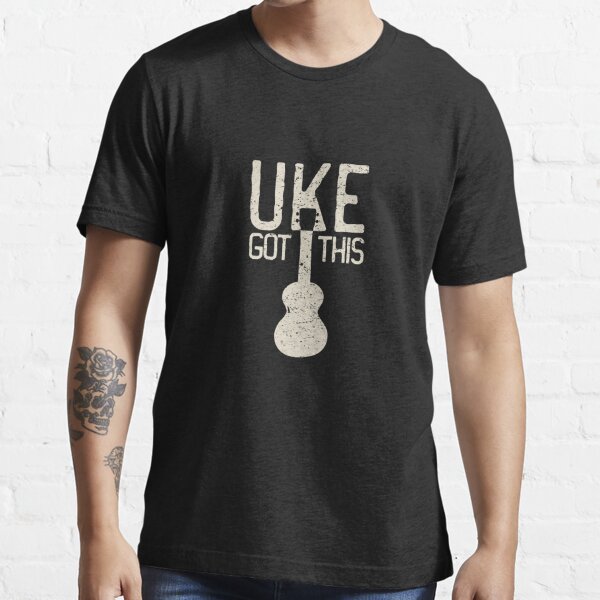An up-close image of a tall male wearing an extra-large black cotton t-shirt, designed with the playful phrase "UKE got this" printed in white. The design incorporates a ukulele silhouette cleverly positioned under the letter K to extend into the word, combining seamlessly with the text "You got this." The man's right forearm displays a detailed black and white tattoo, featuring a skull with a rose and leaves extending from it. Though the man's face is out of focus, he appears to be looking towards his right. The background is composed of a slightly blurred white brick wall, suggesting a casual or urban setting. He is also wearing blue denim jeans, cut very short at the bottom.